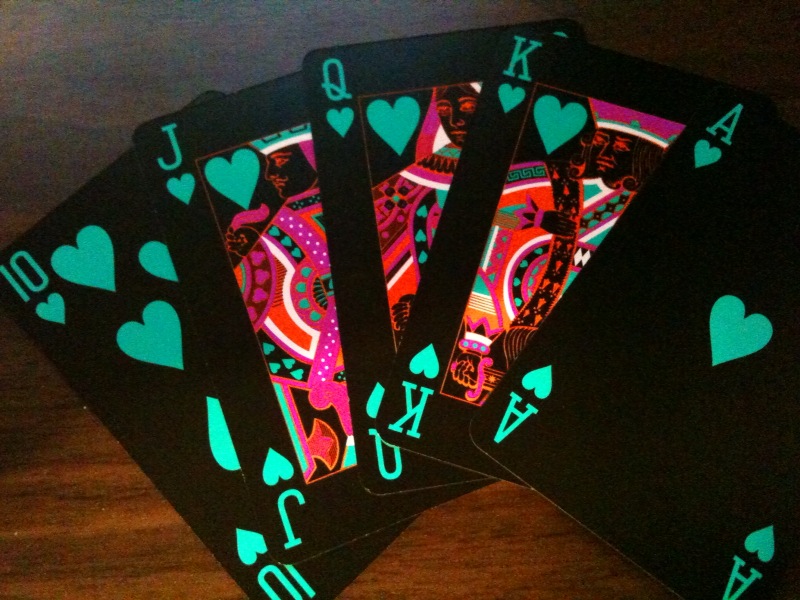The image displays a meticulously arranged hand of playing cards, fanned out across a rich brown wooden table. The composition reveals a royal flush in hearts, showcasing the 10, Jack, Queen, King, and Ace. Unique in design, these cards feature a black background with the suit symbols and numbers in a striking neon green. The Jack, Queen, and King are adorned with modern, high-tech imagery infused with vivid pink and orange shades, lending a futuristic, almost glow-in-the-dark appearance to the cards. This vividly modern aesthetic complements the classic elegance of the royal flush, the highest hand in poker. The scene is devoid of any additional elements, highlighting the distinctive and stylish deck.